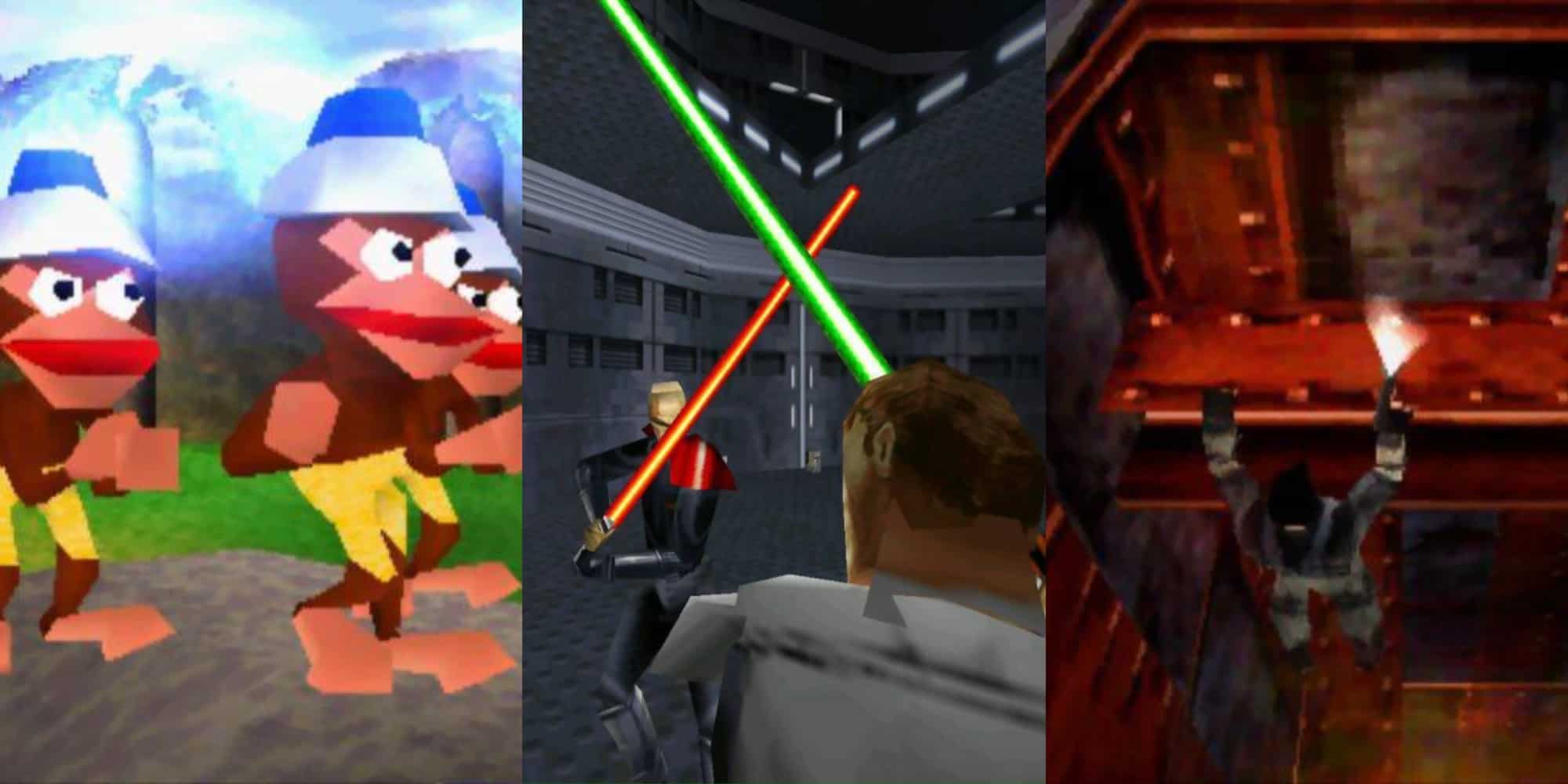The image is a rectangular collage divided into three vertical sections, each showcasing a distinct scene from video games, seemingly from the early 2000s, potentially from the Nintendo 64 era.

The leftmost section features three monkeys standing side by side in the daylight, each clad in yellow shorts and weird white and blue hats. They resemble characters possibly from the game Donkey Kong, all looking in the same direction with a vaguely angry expression.

The central section depicts an intense battle scene with two individuals wielding colored swords reminiscent of lightsabers. The character in the background wields a red lightsaber while wearing a long black outfit, and the one in the foreground sports a white shirt with a green lightsaber. They appear to be engaged in combat within a futuristic, gray-and-black setting, evoking the feel of a Star Wars game.

The rightmost section shows a man garbed in military or spy-like attire, predominantly black and gray, hanging precariously from a red metal beam. The surrounding environment suggests an industrial or warehouse setting, with interconnected steel beams forming the structure around him.